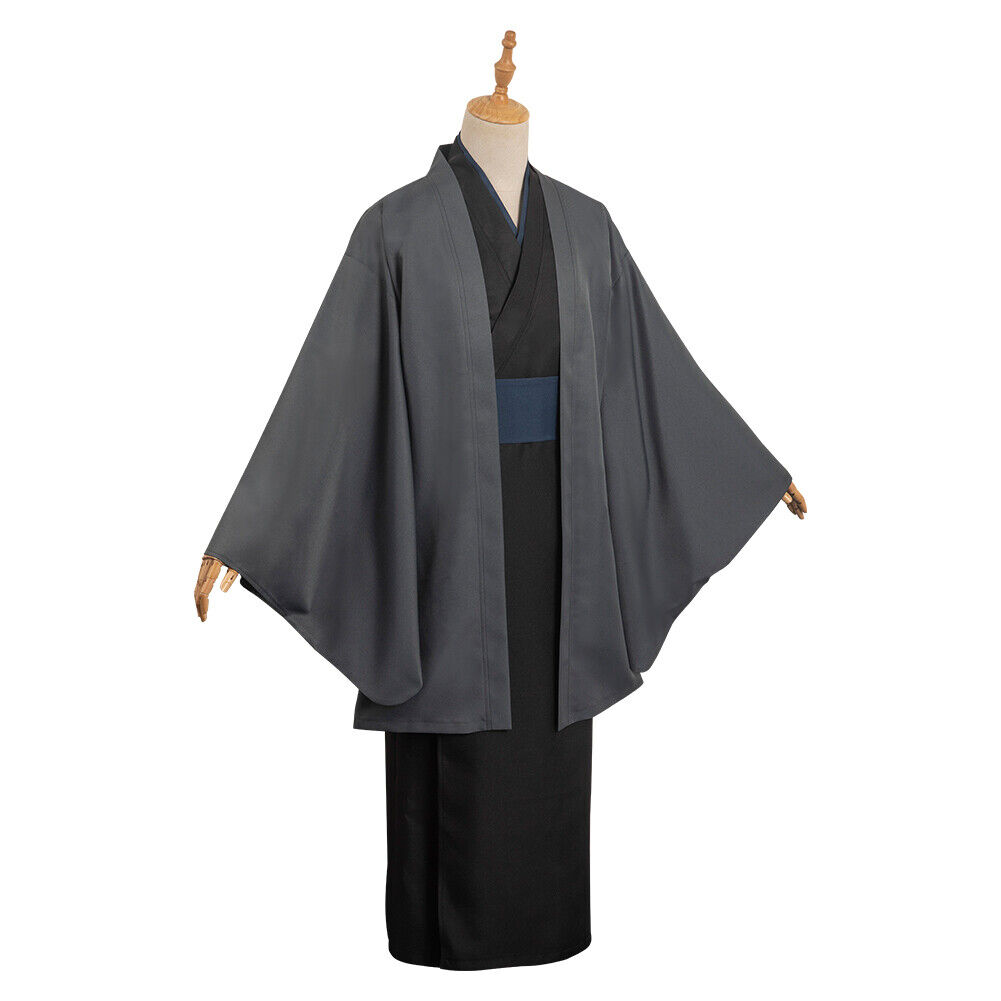This color photograph, presented in portrait orientation, showcases a traditional Japanese outfit displayed on a headless mannequin. The mannequin wears a dark gray cape that extends to the hips, with the arms subtly fanned out to reveal its design, and the hands partially visible at the edges. Beneath the cape, there is a black dress with a knee-length skirt and a crisscross wrap style at the top. Cinching the waist is a dark blue cummerbund-style belt made of fabric. The overall presentation is minimalist, devoid of any ornamental embellishments, embroidery, or additional decorations, emphasizing the comfort and simplicity of the attire. The mannequin is positioned facing the right side of the image, slightly tilted towards the viewer, with a cream-colored neckline and a pointed brown wooden dowel replacing the head. The photograph utilizes representational realism and fashion photography techniques, with the background dropped out to create a floating effect against a clean, white backdrop.